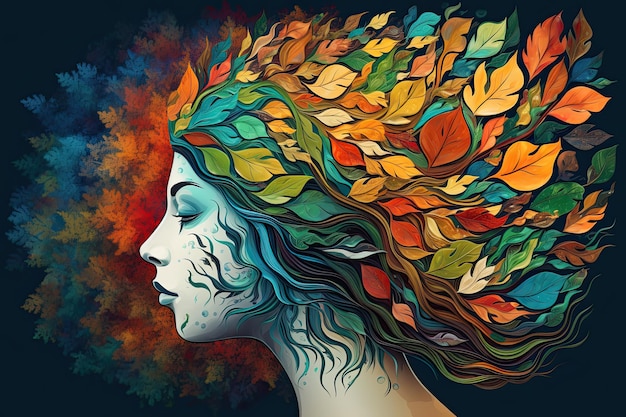This is an intricate, horizontal digital illustration of a woman's side profile, focusing on her head from the neck up. The woman's pale white face, tinged with blue hues around her eyes and lips, exudes a sense of serenity or melancholy. Her face is adorned with artistic, wave-like blue lines. The hair, beginning near her face, gradually morphs into a mesmerizing array of colorful leaves. These leaves, forming a voluminous and flat afro-like structure, feature a spectrum of fall colors—ranging from deep greens and blues to vibrant oranges, yellows, and reds. The strands of her hair appear to be caught in an upward breeze, with leaves flowing and pointing to the right. The background is a rich, dark blue that further accentuates the vividness of the leaves. Overall, this detailed portrayal captures a blend of natural elements and artistic expression intertwined in a single, captivating image.